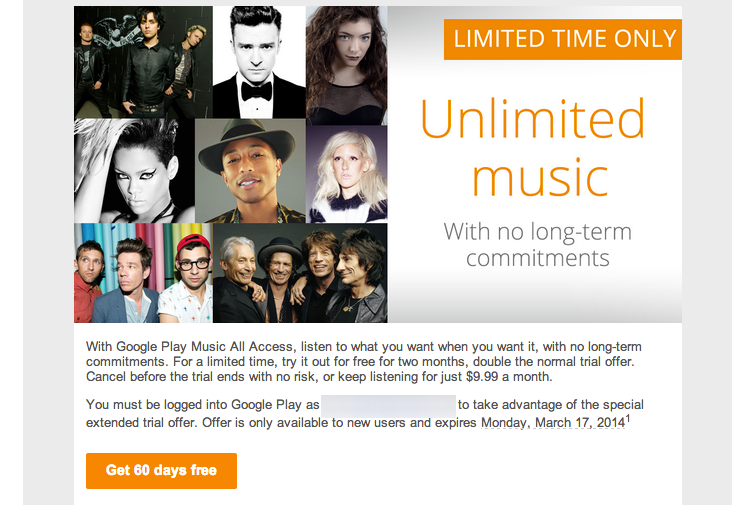The digital advertisement is presented in landscape orientation with a pale grey background, featuring narrow borders on the top and sides. At the top of the ad, there is a section divided into two squares. The right square prominently displays the text "Unlimited Music" in bold orange letters, followed by "with no long-term commitments" in grey. This square also features a striking orange banner at the top saying "Limited Time Only" in white text.

To the left, the square showcases a collage of photographs depicting various musical artists and bands. Starting from the top left, there is an unrecognized artist, followed by a black-and-white photo of Justin Timberlake in a tuxedo. To the right, there's a color photo of Lorde. The second row includes a black-and-white image of Rihanna, an immediately recognizable artist with a hat, and to his right, a blonde artist who is unidentifiable. The bottom row features a photo possibly of Harry Styles, depicting three men in colorful surroundings, and finally, a classic image of the Rolling Stones in their middle-aged years, including Charlie Watts, Ron Wood, Keith Richards, and Mick Jagger.

Below this section, a white rectangle contains the ad's main text in black or grey font. It reads: "With Google Play Music All Access, listen to what you want when you want it with no long-term commitments. For a limited time, try it free for two months." There is an additional note about the trial offer, including a statement: "You must be logged into Google Play as [blacked out name]."

An orange button located at the bottom left of the ad states "60 days free," inviting viewers to take advantage of the offer.